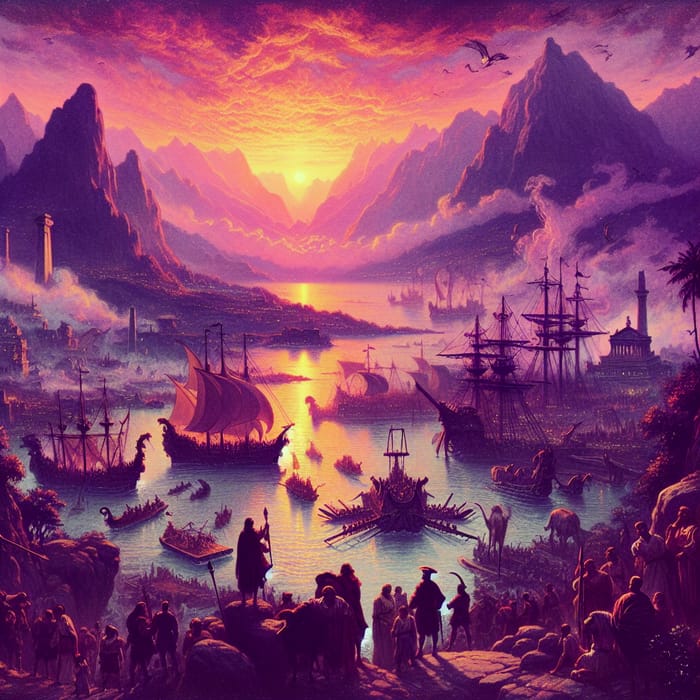This imaginative drawing depicts a fantastical landscape bathed in golden and purple hues. In the sky, amidst a plethora of clouds, tiny dragons soar towards the upper right corner. Nestled below the dramatic skyline, a series of grey, spire-like mountains stretch into the distance, enveloped at their bases by wisps of fog or smoke. Between the mountains, towards the middle-left of the image, the sun shines brightly, creating a striking contrast with the surrounding clouds.

The middle section of the artwork reveals a sprawling bay, crowded unrealistically with various boats, some with raised sails and others without. This congested waterway gives way to a continuation of the bay, extending forward into a larger body of water. On the left side of the image, several towers and buildings dot the landscape, while on the right, additional structures, including a tall tower, rise against the mountainous backdrop.

In the foreground, a rocky expanse slopes down to the water’s edge, where numerous figures are positioned. These people, distinguished by old-fashioned clothing and some adorned with long capes or even a staff, stand gazing out over the water. Among them, an animal, possibly a cow, adds to the scene’s surreal nature. The overall composition, dominated by deep purples and intricate detailing, evokes a sense of otherworldly wonder.